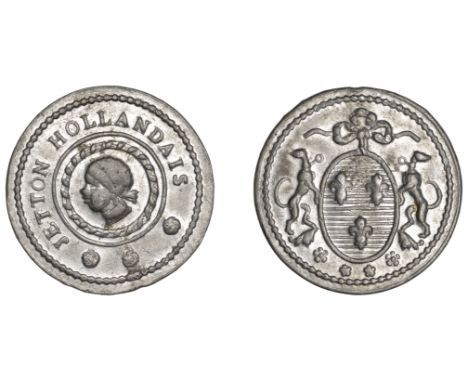This image features two silver coins on a white background, possibly displaying the obverse and reverse sides of the same coin. The coin on the left, which is not particularly shiny, bears the inscription "Jeton Hollandaise" encircling a human profile facing left, adorned with a head wrap or bonnet. This central image is bordered by multiple circles, including a distinctive braided rope design, and three dots separating the words "Jeton" and "Hollandaise." The coin on the right showcases an elaborate design featuring two possibly greyhound-like animals facing each other, standing on their hind legs with their front legs resting on the coin's central crest. This crest comprises three smaller, shield-like shapes. Above the animals is a decorative bow, and below are additional small flowers. Both coins are richly detailed, emphasizing their intricate borders and heraldic elements.